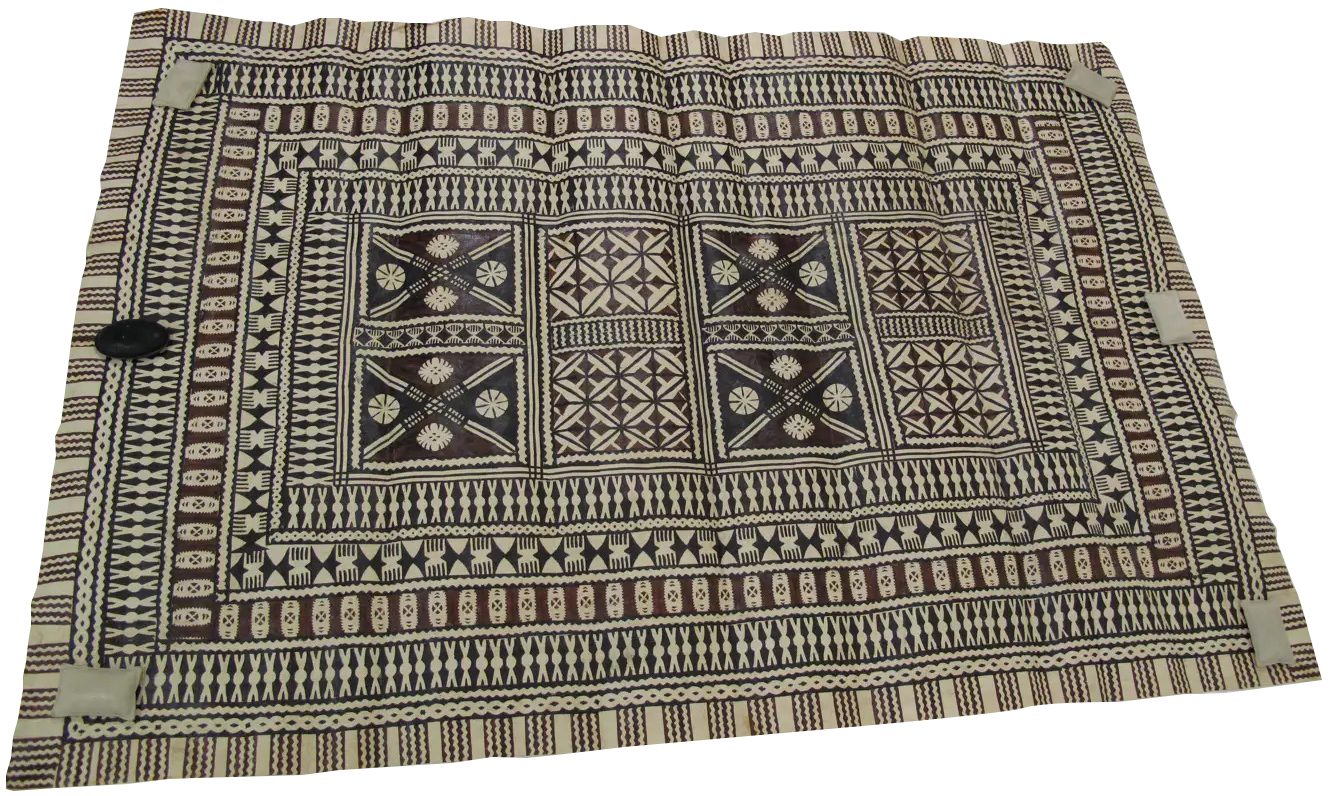The image depicts a richly patterned piece of fabric, possibly a throw blanket, picnic blanket, or even a mat or placemat, displayed against a white background. The fabric features a complex and busy design with multiple geometric patterns in dark colors, such as maroon, dark greens, and dark browns, interspersed with beige elements. The central section of the fabric contains eight distinct square or rectangular blocks, each adorned with decorative motifs including X-shaped designs, floral elements within triangles, and other geometric shapes. The borders of the fabric showcase a simpler pattern consisting of squiggly lines on a beige background. The fabric appears to be weighted down at intervals by small, pillow-shaped pads in beige and a single black circular weight positioned on the left side. The photograph, taken from above, captures the creases and textured details of the fabric, highlighting its intricate and varied design.